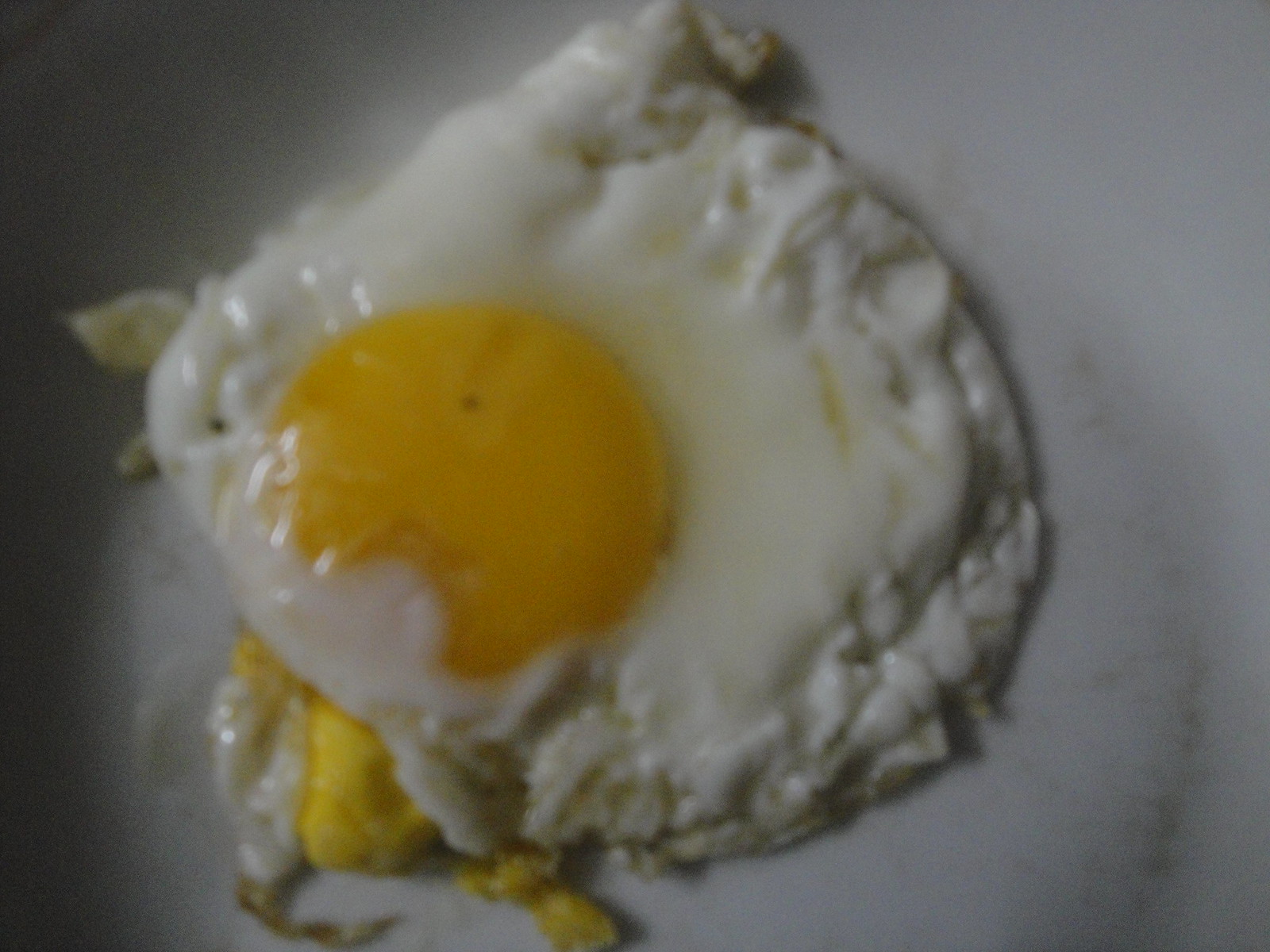This image showcases a fried egg, possibly resting on a white plate, though the surface beneath, appearing gray, remains ambiguous and could potentially be a nonstick pan. The egg itself exhibits an unevenly cooked texture, highlighted by a rough, slightly crispy brown edge. The whites extend outward, displaying a few cooked but not overly runny areas, specifically where a portion spills out from underneath. The yolk, predominantly dark yellow with a slight half-moon misshapen indentation on the bottom left side where white overlaps, is indicative of an imperfect but well-cooked egg. Notable details include a black speck about a third of the way down the yolk, and a couple more black specks in the whites nearby. The overall appearance suggests an egg that, while not perfectly formed, is still adequately prepared and ready to eat.